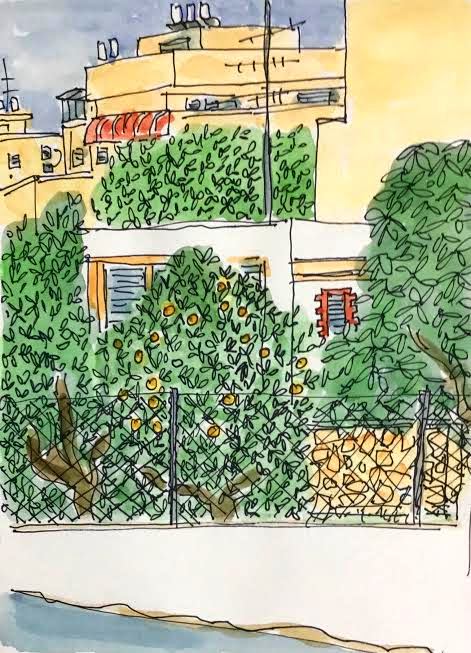A vibrant urban scene captured in black ink and fine-point marker, later brought to life with watercolors. The scene showcases yellow or sand-colored buildings, complemented by tall bushes or possibly orange trees, one notably featuring a trunk with round, orange fruit. The sky appears troubled, hinting at a stormy day, yet no rain falls. The flat-roofed structures suggest a typically dry climate. In the foreground, a chain link fence sits atop a white concrete barrier, beyond which three trees stand, one abundant with oranges. A striking white stucco building with yellowish-orange trim and red shutters, its windows covered in Venetian blinds, adds character. Behind this building, another tree emerges. Taller sand-colored buildings with flat tops, telephone poles, and rooftop antennas populate the background. In the lower left-hand corner, water flows by, reflecting what might be a canal or drainage system.